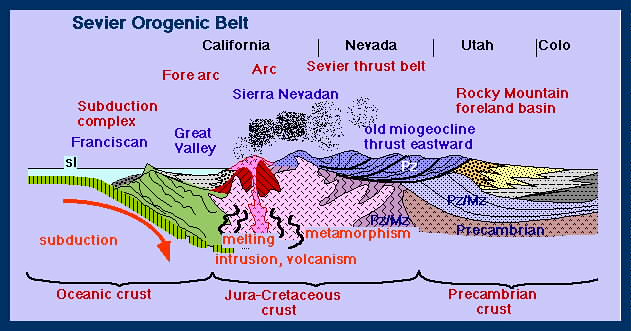This detailed image is a comprehensive chart illustrating the Sevier Orogenic Belt, focusing on the geological breakdown of Earth’s crust from the coastline to various inland regions. It spans from California to Colorado, highlighting significant geological areas and processes. The chart, rectangular in shape with blue and purple borders, prominently labels key regions: California, Nevada, Utah, and Colorado. The diagram details distinct crust layers at the bottom - Oceanic Crust, Jura Cretaceous Crust, and Precambrian Crust - and emphasizes geological features such as the Subduction Complex, Fore Arc, Arc, and Sevier Thrust Belt. The land divisions are marked with names like Franciscan, Great Valley, Sierra Nevada, Old Mio Geocline, and Rocky Mountain Foreland Basin. Various colors like green, blue, and yellow signify different layers and areas, with additional elements such as mountains and arrows indicating direction and movement of the earth plates. This visual representation serves to explain the geological strata and dynamic processes shaping these regions.